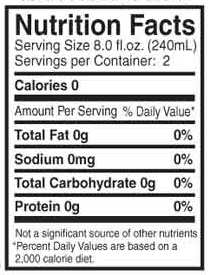A slightly blurred image of a nutrition label set against a white square with a black border. The text reads "Nutrition Facts" at the top, followed by details including "Serving Size: 8 fluid ounces." The blurriness of the image makes some of the text difficult to read, but the essential information about serving size is discernible.